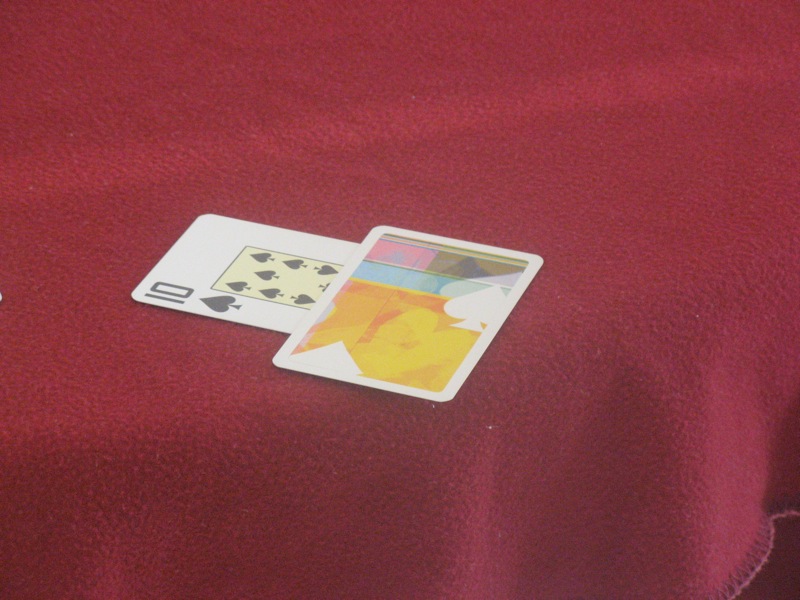This photograph features a textured red tablecloth that resembles felt, giving it the appearance of a well-loved blanket. The tablecloth shows signs of wear, with visible pills indicating it has been frequently washed and dried. At the bottom of the tablecloth is a sewn thread pattern in a shade of red that closely matches the fabric. The cloth is draped over a table, though the table itself is not visible, only suggested by the shape of the draped fabric.

On top of the tablecloth, there are two playing cards placed near each other. The card on the left is positioned horizontally and displays the ten of spades, identifiable by its black spade symbols. The card on the right is oriented more vertically, though slightly tilted, and its back shows a colorful design. This design includes a yellow splotch, a blue rectangle, a small pink square, and a silhouette of a white spade in the center.

This arrangement of the tablecloth and playing cards creates a cozy and detailed scene, evoking a sense of casual leisure or a momentary pause in a game.